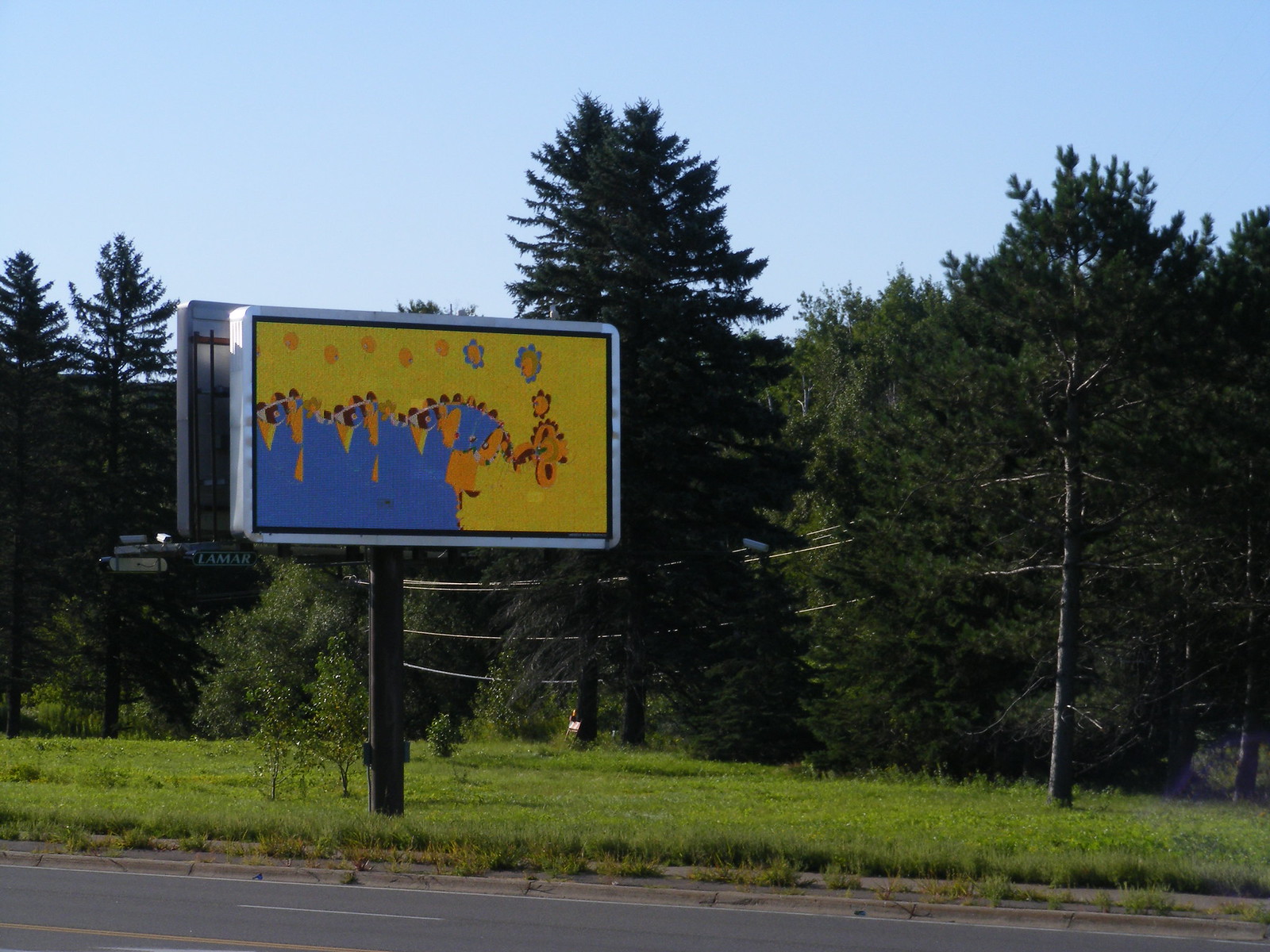The image captures an old billboard situated on the side of the road, prominently mounted on a thick, black, cylindrical pole. The billboard is rectangular and displays a partially peeled-off advertisement, showing a patchwork of yellow with scattered orange splotches and a blue section in the lower right-hand corner. The remnants suggest layers of previous ads or perhaps an attempt at painting over it. The bottom left corner of the billboard bears the name "Lamar," indicating the brand of the billboard.

Surrounding the billboard is a lush, green field of grass approximately a foot tall, interspersed with two small trees. In the background, dense evergreen trees stretch towards the top of the image, set against a clear blue sky, framing the billboard. At the bottom of the image, a grey asphalt road with white dotted lines and solid double yellow lines indicates the proximity to a highway, suggesting that the photo was taken from across the street. The scene emphasizes the juxtaposition of the natural elements with the weathered, industrial appearance of the billboard.